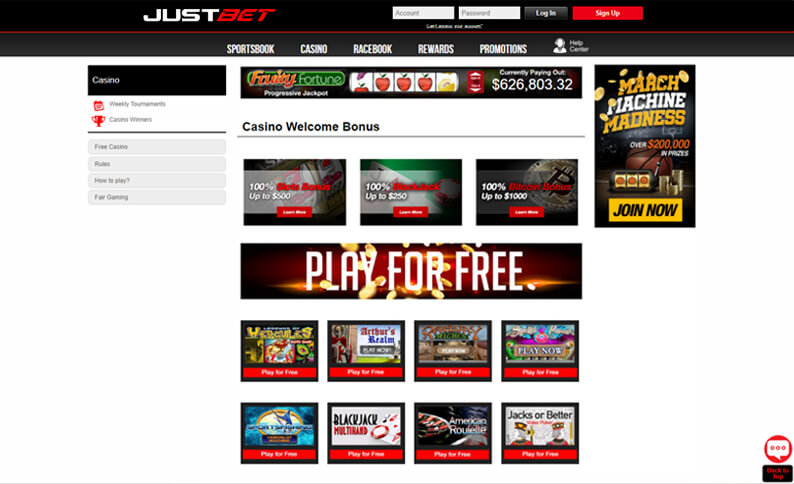This is the front page of a website, centered around the "Just Bet" logo in bold white text. The word "Just" is in a regular font, while "Bet" is italicized and highlighted in red. Two fields for user input are prominently displayed below the logo: one for the account name or number, and another for the password, which appears slightly blurred. To the right, there is a black "Login" button and a red "Sign Up" button, all contained within a black strip separated by a red line.

Below this, a navigation bar offers various options: "Sportsbook," "Casino," "Race Book," "Rewards," "Promotions," and a user account icon. Dominating the main part of the page is an image of a slot machine featuring a single row with five symbols and an adjacent symbol. Above this is a large dollar amount—$626,803.32—indicating a possible jackpot or prize.

Beneath this, the text "Casino Welcome Bonus" appears alongside several eye-catching images. The phrase "Play for Free" is prominently displayed in the center of this section. On the right-hand side of the page, there is a promotional banner for an event named "Machine Madness," featuring a call to action: "Join Now," positioned next to a vibrant image.